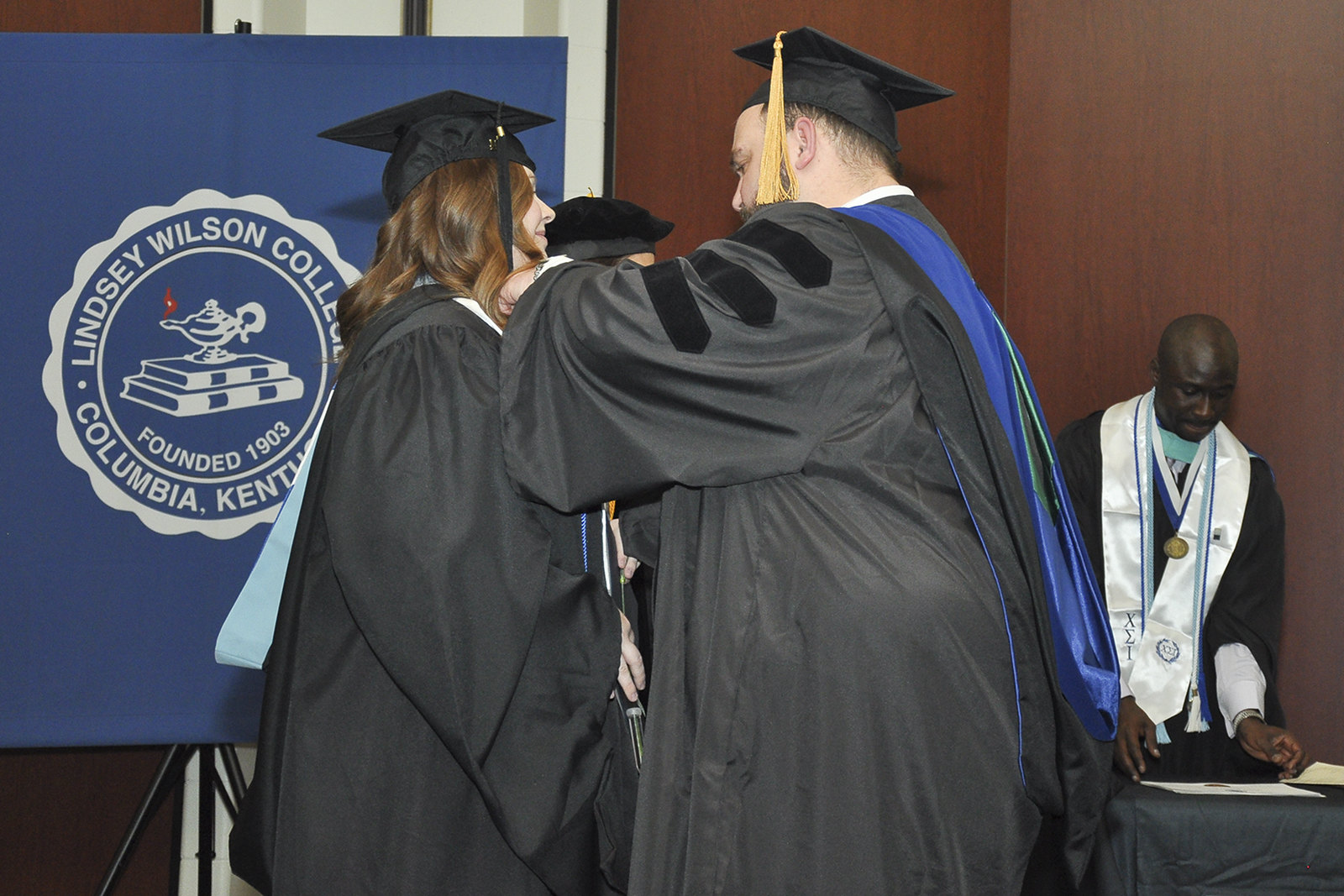This detailed image captures an indoor graduation ceremony featuring several individuals. Dominating the foreground are two figures: a woman on the left with long, thin brown hair under a black graduation cap and gown with a light blue ribbon down her back, and a man on the right with black hair wearing a black cap and gown adorned with a blue sash. He has a gold tassel on his cap and is reaching out with his hands, seemingly adjusting something around the woman's neck.

In the background on the right-hand side, there's a bald African-American man dressed in a black graduation gown with a white sash draped around his neck. He also wears a medal hung by a blue and white string. Further enriching the scene is a dark wood-colored wall on the right and a prominently displayed blue poster on the left. This poster features a white circular logo that reads "Lindsey Wilson College, Columbia, Kentucky," with a lantern perched atop a stack of books at its center, and notes the founding year, 1903. The style of this photograph is representational, capturing a realistic depiction of the graduation moment.